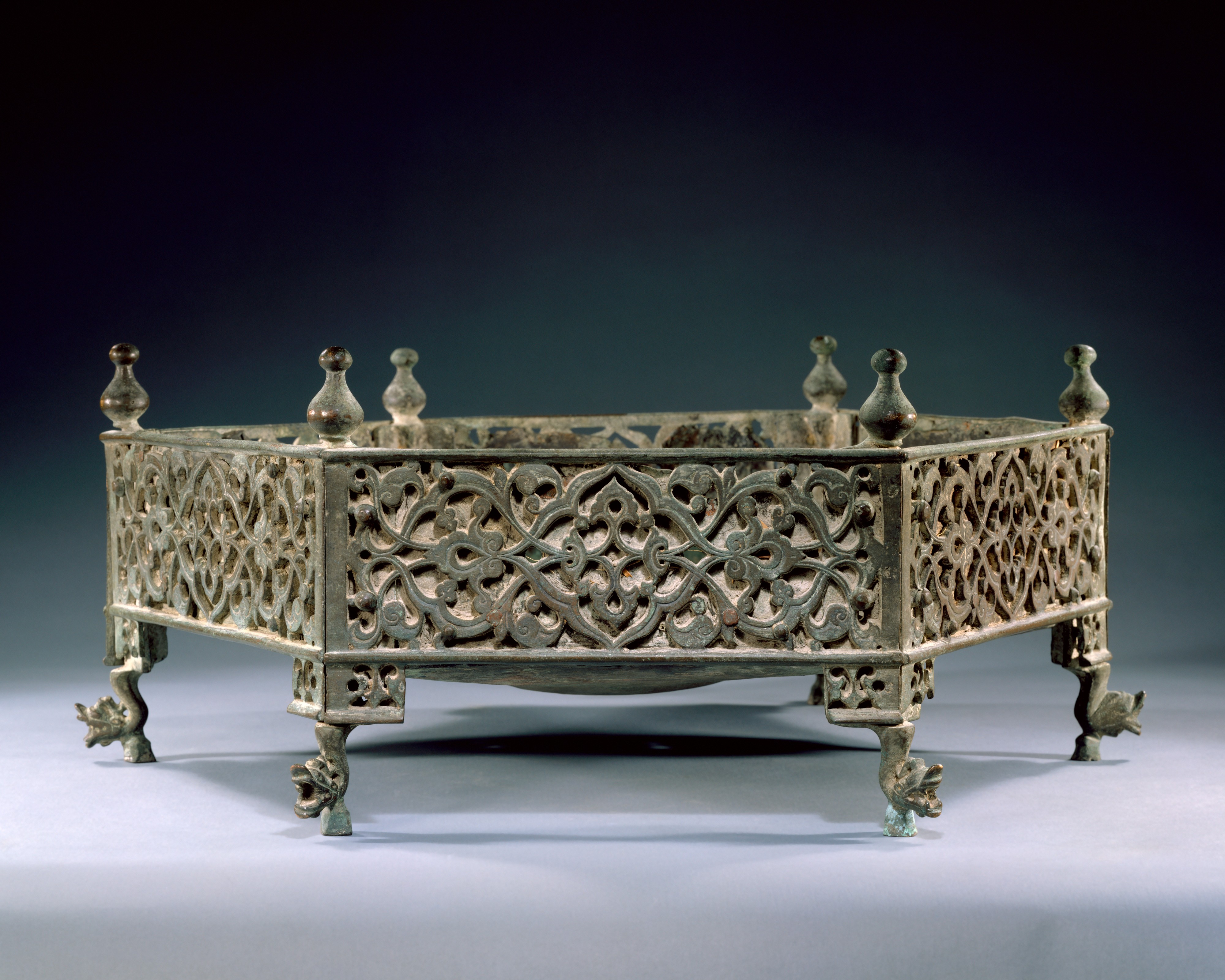The image displays an intricately designed, hexagonal metallic tray, standing on six legs, each adorned with a dragon head at the base. The tray appears aged, with traces of chipping paint revealing its former silver glory. Its sides and the inner platform are bordered by elaborate patterns resembling leaves or flowers in black and silver. At each corner of the tray's top rests a structure shaped like a basketball with a round knob, reminiscent of chess pawns. The tray casts a shadow on the white surface it stands upon, while the background gradually transitions from black at the top to lighter shades of grey towards the bottom.